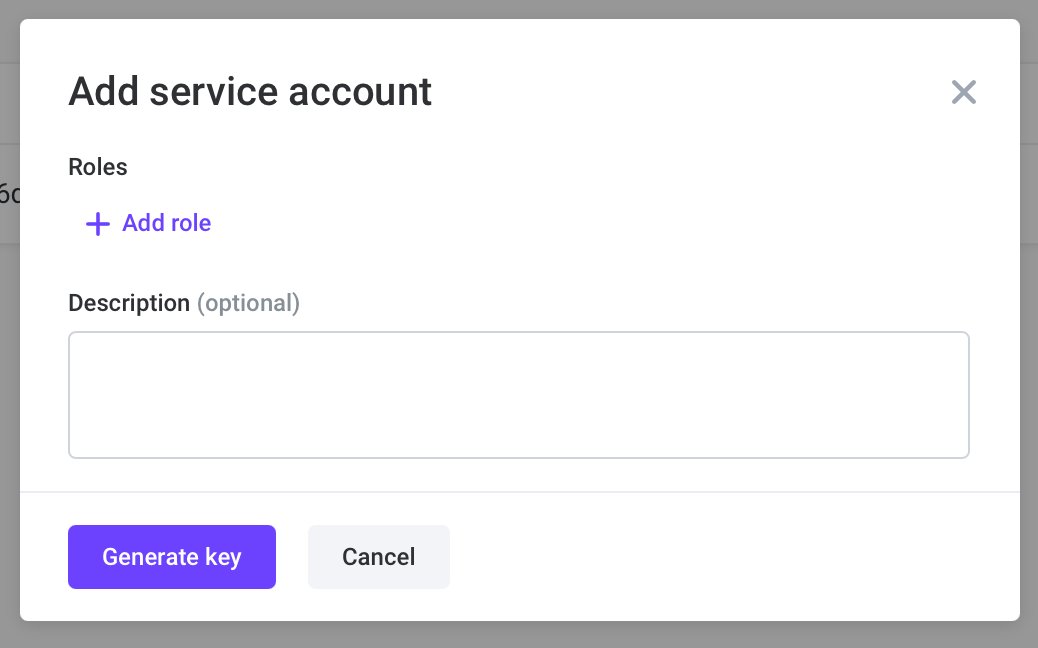The image displays a small pop-up window from a website with the heading "Add Service Account." The overall background of the image is gray, while the background of the window itself is white. In the top-right corner of the window, there is a small "X" icon for closing the pop-up. 

The content within the window starts with the heading "Add Service Account" on the extreme left in black text. A few spaces to the right, in smaller font, the word "Roles" is displayed. Farther to the right, there is purple text that reads "Add Role," preceded by a plus sign. Continuing to the right, the text "Description" is in black, followed by "optional" in parentheses and colored gray.

Below this section, there is a large horizontal rectangular text box for entering the description. Directly under this text box, a thin horizontal line separates the elements within the pop-up. Beneath this line, there are two buttons positioned to the left. The first button, labeled "Generate Key," is purple with white text, and the second button is gray, labeled "Cancel" in black text.